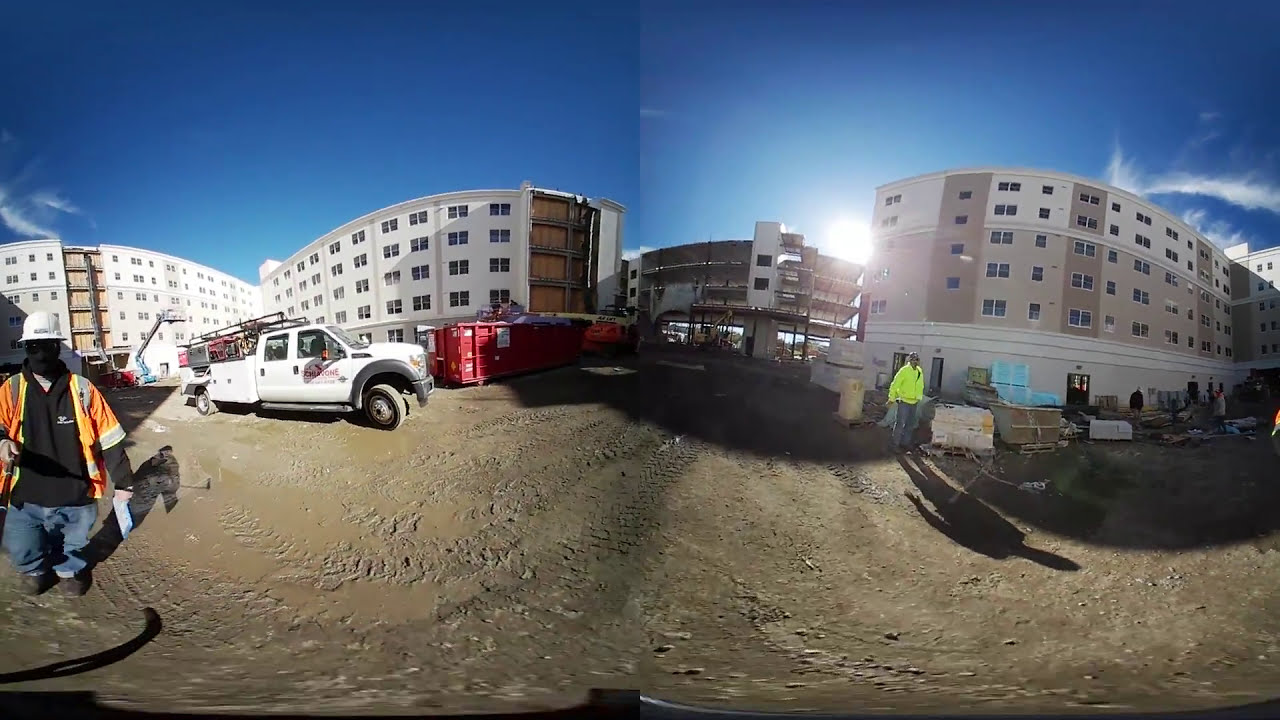The image depicts a bustling construction site of a large apartment complex, captured with a fisheye lens, giving it a slightly distorted, panoramic view that almost looks pieced together down the center. The main building complex, predominantly white and reaching about four to five stories high, stands prominently with many square windows. Adjacent to it is a tan and brown building with similar square windows. Scattered around the site are multiple pallets stacked with various construction materials and red storage containers possibly being used as garbage bins.

In the foreground are several construction workers, clad in high-visibility vests and hard hats, moving about the area. On the left, a man in an orange vest, black shirt, jeans, and an orange helmet is partially cut off but noticeable; he appears to be carrying a piece of paper. Further left, another worker in a black mask, white hard hat, orange jacket, black shirt, and jeans is seen standing. To the right, a worker in a bright yellow jacket and helmet stands in front of a pallet stacked with stone blocks. A white construction truck is parked nearby on a dirt path marked with tire tracks. The vivid blue sky and shining sun indicate it's daytime. Although the scene is tinged with a blend of debris and dirt, construction activities continue under the clear, sunny sky.